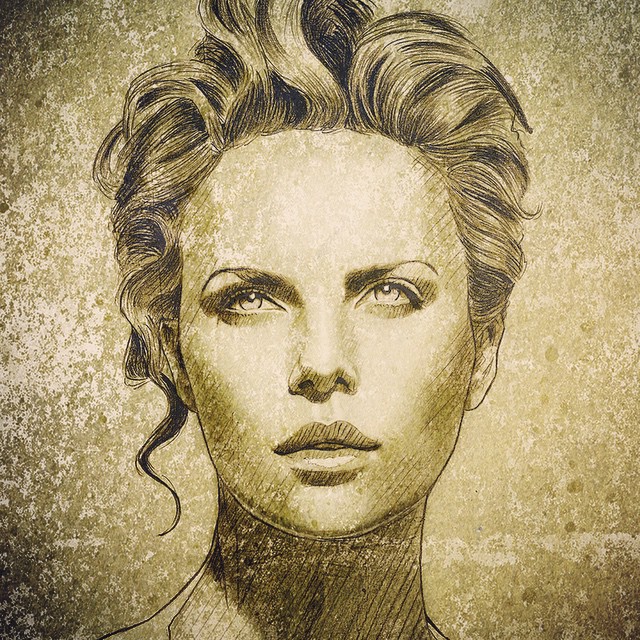This is a beautifully detailed drawing of a woman resembling Charlize Theron, the renowned actress from South Africa. Rendered in shades of brown and bronze, the artwork showcases a serene and thoughtful expression on her face. Her short, wavy hair is either pulled back or styled high on top, with a single tendril dangling elegantly on her left side. The background mirrors the golden and bronze hues of her complexion and hair, featuring a splotchy pattern that enhances the overall harmony of the piece. Her features are meticulously detailed: rounded eyelids, a refined nose, and a full, expressive mouth. She gazes upward and to her right, and her long neck displays meticulous diagonal hatching, adding depth and texture to the drawing. The entire image radiates professionalism and elegance, capturing the serene beauty of the subject in a strikingly minimalist yet profoundly evocative manner.